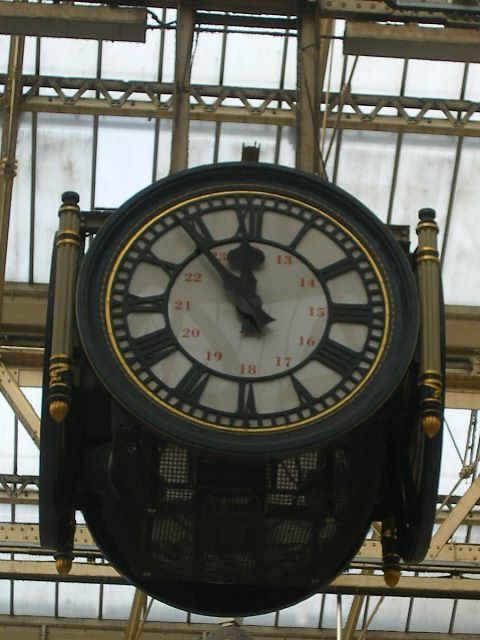The image showcases an expansive room, where both the ceiling and walls are dominated by an array of large windows. The windows, framed in brown and metal, feature elongated rods descending from the ceiling. Although the windows stretch into the distance, their frosted surfaces obscure any view beyond them. Prominently positioned in the foreground is a striking round clock. This clock, composed of black metal, is encased in a cage-like framework. Flanking the clock are two brown and gold wooden pieces that add to its elegant framing. The clock's face is a pristine white, adorned with black hour and minute hands, and marked by Roman numerals. A gold rim encircles the clock face, adding a touch of gleaming detail to its sophisticated design.